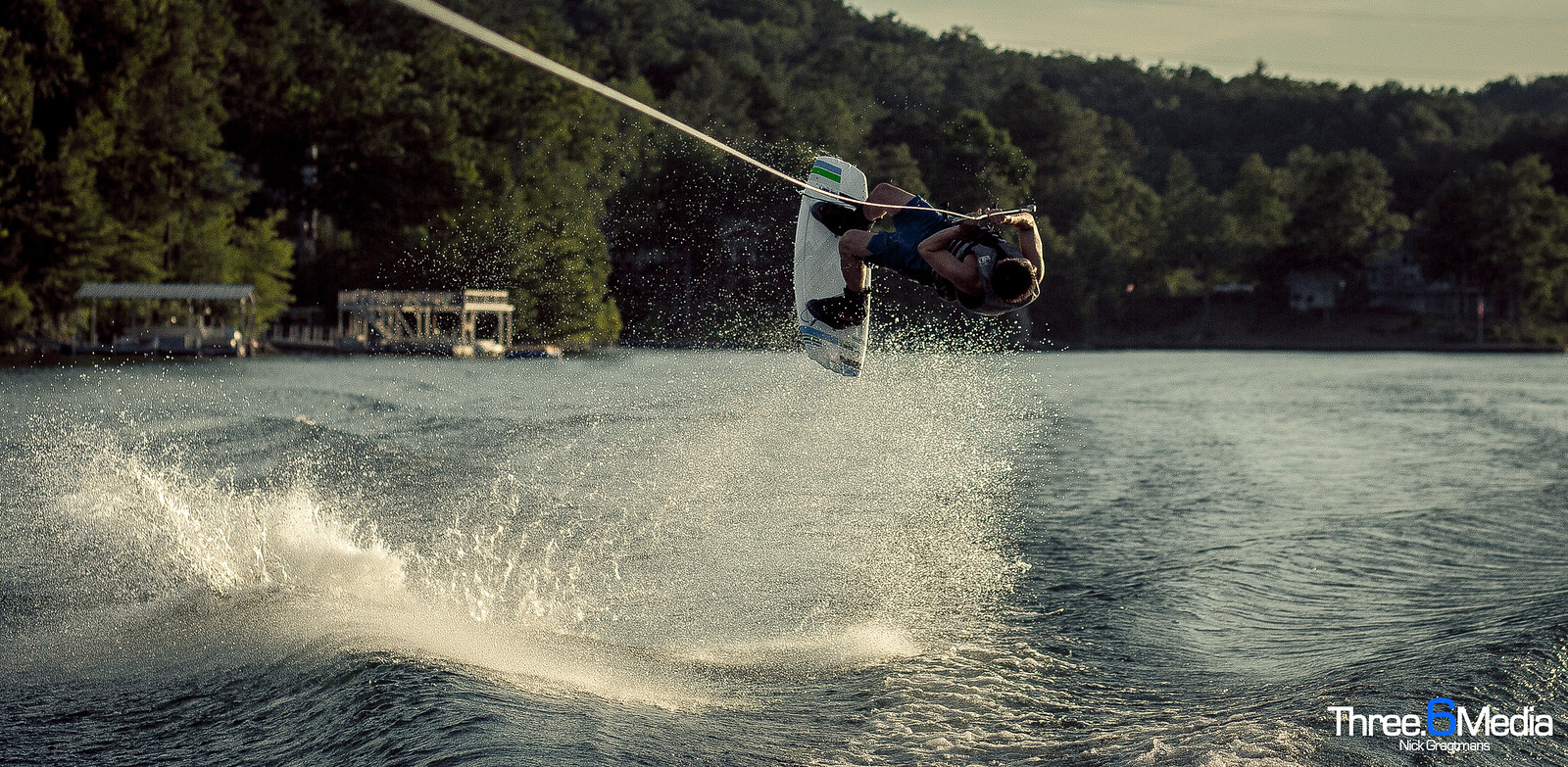In this panoramic image, we see a large, vibrant lake surrounded by trees and boathouses. The main focal point is a male wakeboarder, estimated to be in his 20s or 30s, performing an aerial stunt high above the water. The rider is captured mid-air, almost horizontal at a 180-degree angle, suspended after tackling a significant wave. He is equipped with a floating vest and black foot gear, firmly strapped to a white wakeboard adorned with green and blue stripes. In his hands, he holds onto a rope connected to the towing boat. The scene suggests a late afternoon setting, with softer sunlight casting hues of greens, blues, and foamy whites across the landscape. The watermark "3.6 Media" along with the name "Nick Gregor Mars" appears in the bottom right corner of the image, with the number '3' in white and '6' in blue. In the distance, two small buildings and multiple ferry boats further enrich the scenic backdrop.